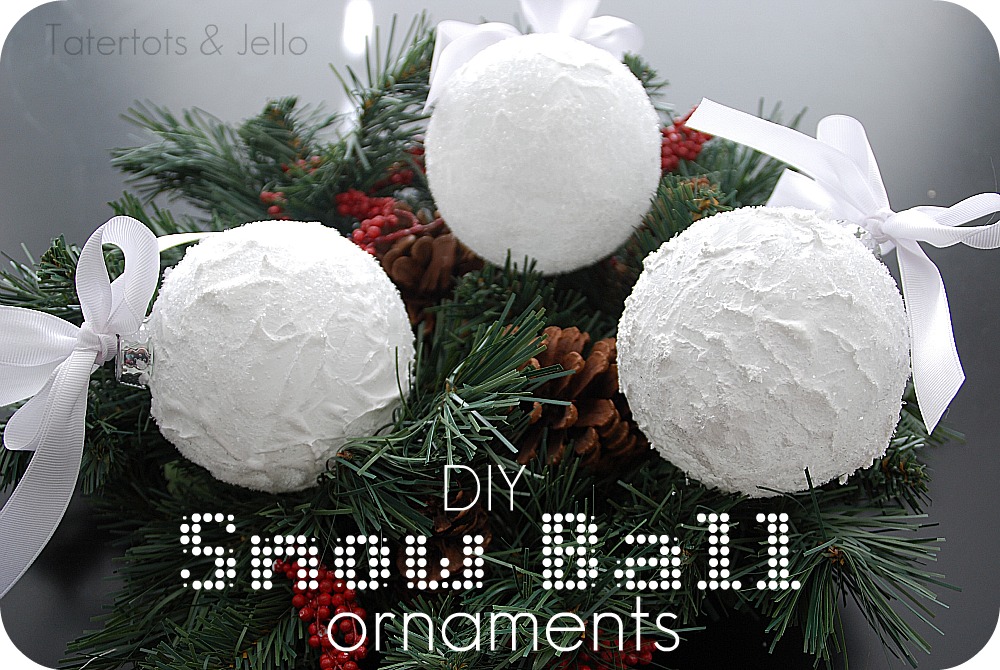This festive image advertises a blog or instructional website and features a meticulously crafted Christmas decoration. Dominating the photograph is a small garland or wreath made to mimic pine tree branches, complete with intertwined faux pine cones, mistletoe, and small red berries. Centered on this lush green foliage are three large, spherical ornaments that are textured to resemble freshly packed snowballs. Each snowball ornament is adorned with a large white ribbon tied elegantly at the top. In bold white text at the bottom of the photograph, the phrase "DIY Snowball Ornaments" invites viewers to create their own holiday decorations, while in the semi-transparent grey text at the top left corner, the name "Tater Tots and Jello" hints at the creative source of this charming holiday project. The rich palette of Snow White, green, brown, red, and subtle greys and blacks enhances the overall festive appeal.